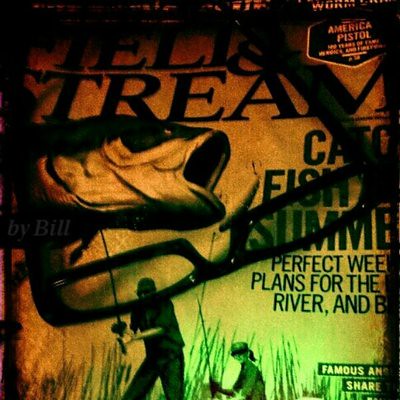The image resembles an old, slightly blurry cover of a fishing magazine, potentially "Field and Stream." It features a detailed drawing of two people wearing baseball caps and sunglasses, fishing in a grassy field. They hold up fishing poles with a very large fish prominently depicted in front of them. The foreground is dominated by a pair of black eyeglasses resting on the magazine cover, obscuring parts of the text. The title appears to say something like "Catch Fish This Summer" and mentions "perfect weekend plans for the river," although much of the text is partially covered or unclear. The magazine's colors are green at the bottom transitioning to orange at the top, adding to the vintage feel of the image.